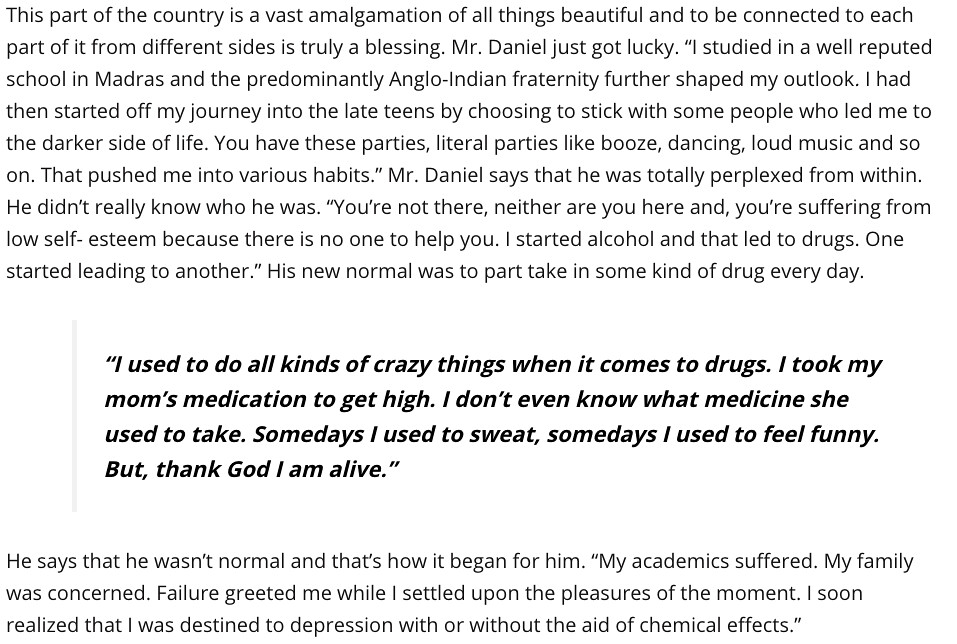The image appears to be an excerpt from a book or webpage featuring a narrative about Mr. Daniel and his experiences with alcohol and drug addiction. The text is primarily a white background with black font. It features several text blocks, including a central bolded quote: "I used to do all kinds of crazy things when it comes to drugs. I took my mom's medication to get high. I don't even know what medicine she used to take. Some days I used to sweat, some days I used to feel funny, but thank God I am alive."

The passage begins by describing the beauty of a particular country and mentions Mr. Daniel's past. He shares memories of attending a reputable school in Madras and being influenced by an Anglo-Indian community. His life took a darker turn in his late teens when he started attending parties filled with booze, dancing, and loud music, leading to substance misuse. Mr. Daniel describes feeling perplexed and suffering from low self-esteem, stating, "You're not there, neither are you here, and you're suffering from low self-esteem because there's no one to help you. I started alcohol and that led to drugs. One started leading to another."

He details how substance abuse became his "new normal," severely impacting his academics and concerning his family. Despite the turmoil, he acknowledges his survival: "Failure created me while I settled upon the pleasures of the moment. I soon realized that I was destined to depression with or without the aid of chemical effects."